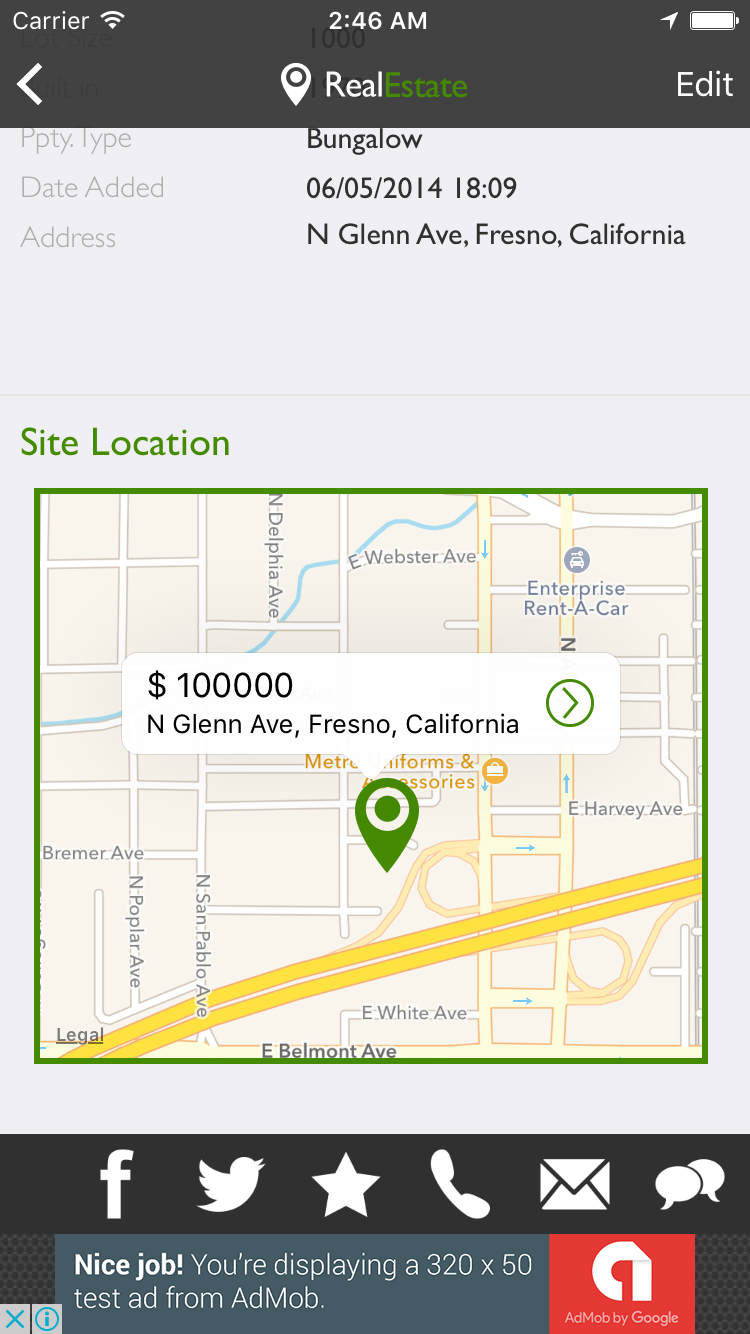This image is a screenshot of a real estate app displayed on a smartphone at 2:46 a.m. The app's logo is prominently featured at the top center of the screen, with the text "Real Estate" divided into two colors: "Real" in white and "Estate" in dark green. Adjacent to the logo on the left is a white location marker icon. 

The top right corner of the screen shows a fully charged battery symbol. Below this, the app displays detailed information about a property. 

The property type is listed as a "Bungalow," and the date added is recorded as June 5, 2014, at 6:09 p.m. The address provided is North Glen Avenue, Fresno, California. Additionally, there is a map section that highlights the property's location and lists the price as $100,000. The map indicates nearby landmarks, including an Enterprise Rent-A-Car location and Metro Uniforms and Accessories.

At the bottom of the screen, there is an advertisement or notification from AdMob, stating: "Nice job! You're displaying a 320 by 50 test ad from AdMob."